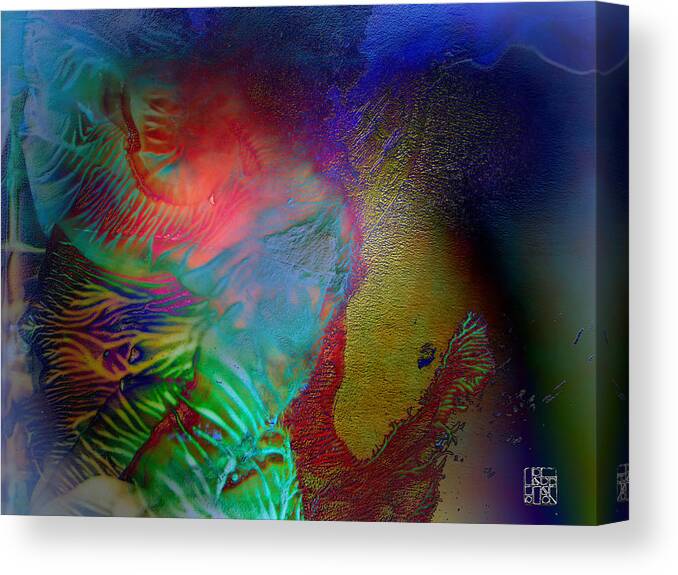This is a photograph of a vivid and intricate canvas painting, showcasing a mixture of acrylic or oil paints with bright, bold colors across the spectrum. The painting is three-dimensional, revealed by the beveled edges visible along the right side. Predominantly abstract, it features a variety of swirling shapes and colors that resemble an underwater scene, with blues and greens evocative of coral reefs. In the upper section, hints of a human face and shoulder emerge amid pink hues, suggesting a human figure. The right side of the canvas is dominated by a golden-yellow that fades into deep purple, adorned with a red and blue diamond-like shape. The artwork is further embellished with red swirls and yellow vein-like shapes scattered against a blue backdrop, with colors blending into quadrants and lines creating a topographical map-like appearance. A notable detail at the bottom right of the canvas is a small white logo or symbol, composed of squares, rectangles, and circles, contrasted against a dark purple background.